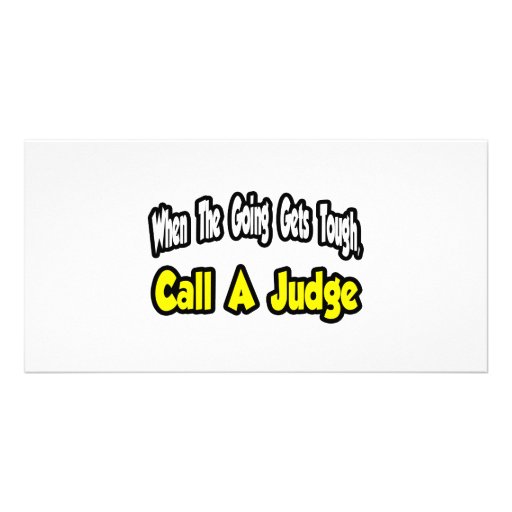The image appears to be a graphic design for a sticker with a clean, off-white background. At the center of the sticker, there is a boldly styled text in two lines: the first line says "When the going gets tough" in white font with a thick black outline, and the second line says "call a judge" in yellow font, also with a thick black outline. The overall design is simple yet striking, making the text stand out vividly against the light background. It's likely intended for humorous use, potentially appealing to a demographic that enjoys playful or rebellious themes, such as skaters or "bad boys." The rectangular design ensures the text is perfectly centered, enhancing its visual appeal for use as a bumper sticker or possibly a greeting card for those familiar with or appreciative of the judiciary.